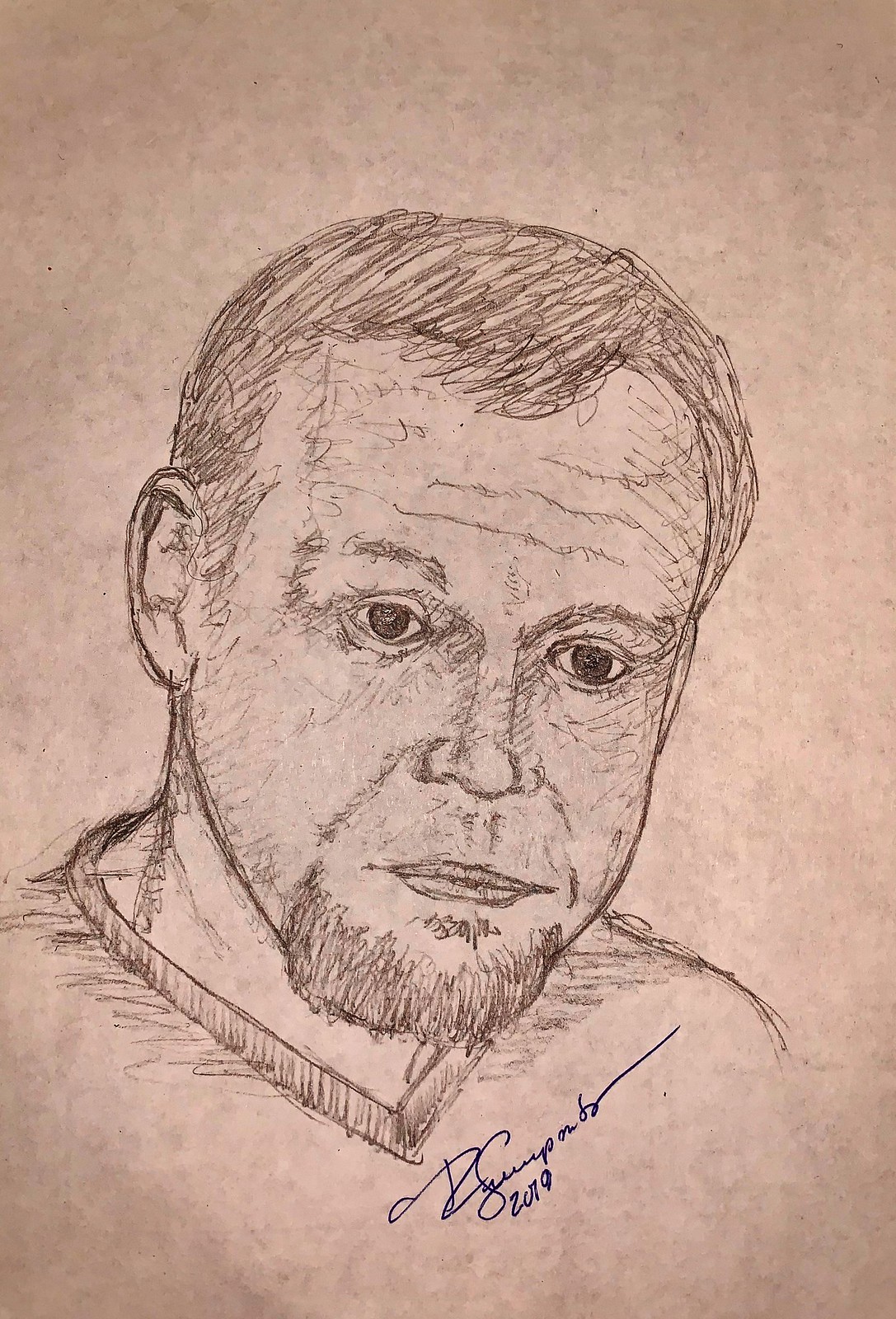This is a detailed line drawing of a young man with short, nicely groomed hair and a well-trimmed beard, including a thin mustache around his nose, a goatee under his lip, and covering his chin. His expression is focused, with lips pressed slightly together, giving him an alert, intent look. He has dark-colored eyes and his head is slightly tilted towards the lower right corner of the portrait, causing his right ear to be visible while his left ear is out of view. He is depicted in a ribbed collar v-neck shirt, with the artist’s signature appearing at a 45-degree angle under the v-neck, rendered in blue ink and dated 2019. The sketch is done on tan-colored paper, with the dimensions covering most of the page and showing his head and the upper part of his chest. The ink used for sketching appears to be dark brown.